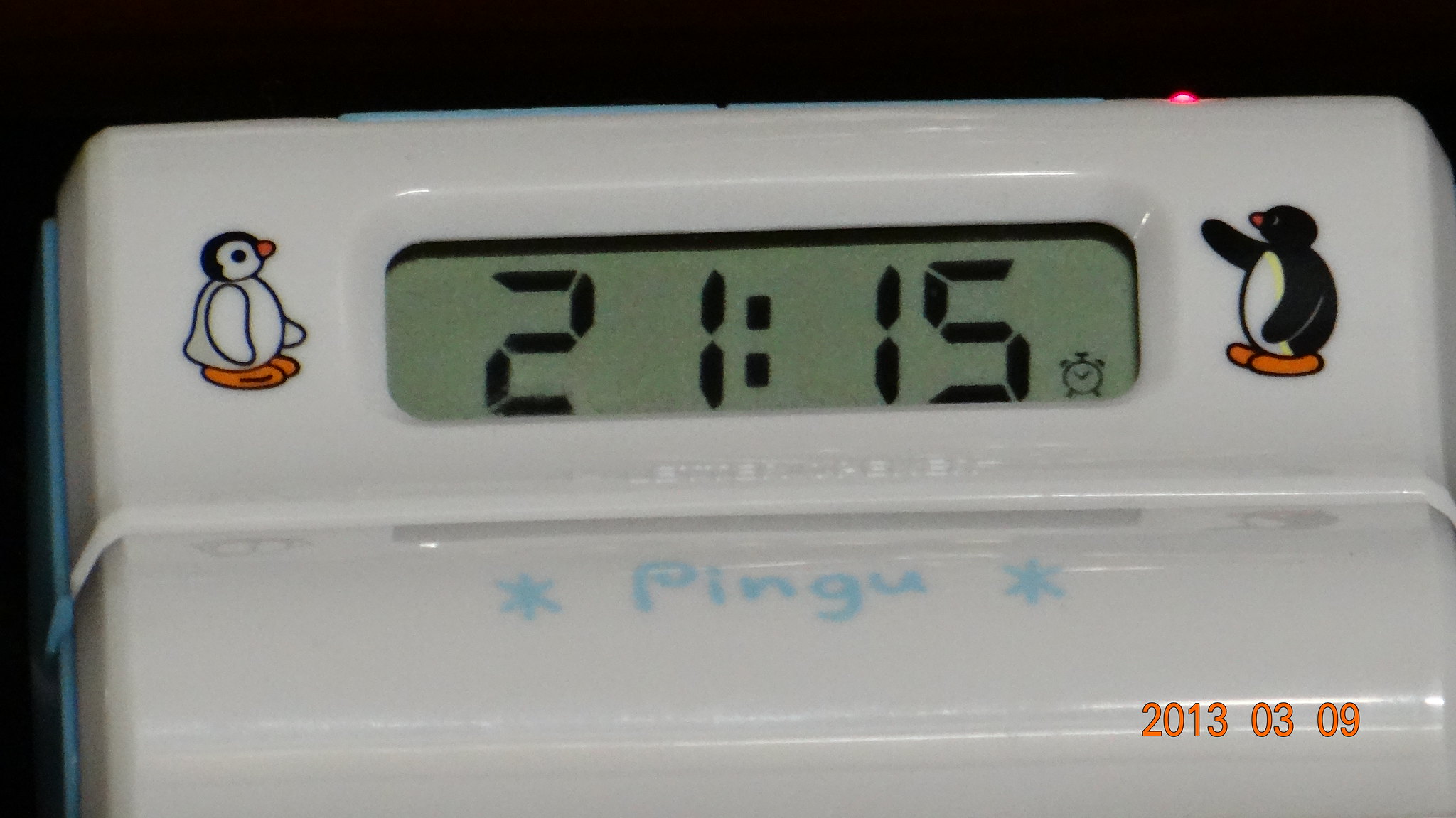This rectangular image features a predominantly white timer or clock, oriented with its longer sides stretching left to right. Central to the device is a digital display indicating "21:15" in bold black numerals, accompanied by a small alarm clock icon situated on the bottom right of the display. Flanking this digital readout are two distinctive penguin figures. The penguin on the left has a predominantly white body with only a minimal amount of black on its head, while the penguin on the right is mostly black, save for a white belly. Both penguins sport bright orange beaks and feet. Directly beneath the display, the name "Pingu" is inscribed in light blue text, flanked by light blue asterisks on either side. In the bottom right corner of the photograph, an orange date stamp reads "2013-03-09."